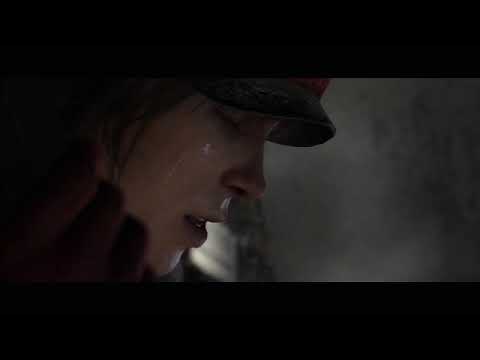The image displays a close-up of a woman's face, prominently positioned towards the left side of the frame with her head tilted down to the right. She appears to be crying, as her wet face glistens with tear stains. A single tear can be seen streaming down her bright white cheek. Her eyes are nearly closed, and her mouth is slightly open, revealing pink lips. She has long black hair, made stringy and clumped together by the rain. The woman wears a dark hat with a small, visible black brim, and a black-colored coat around her neck.

In the bottom third of the image, black widescreen bars stretch horizontally, while a gray, concrete-like wall occupies the background on the right side. From the lower left, a gloved hand clenched into a fist — covered by a burgundy red glove — is faintly visible near her face. The image captures a moment of poignant emotion, emphasizing her soaked appearance and soft, sorrowful expression.